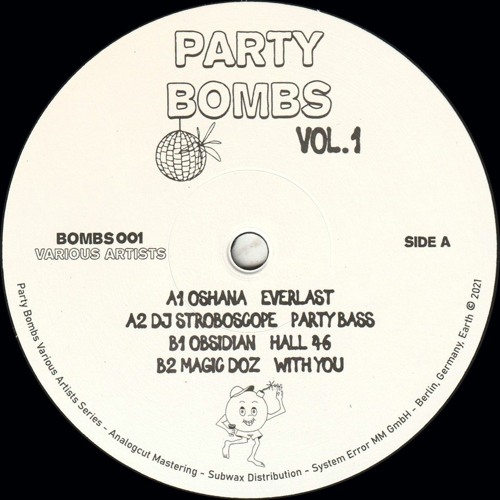This image is a detailed photograph of a vinyl record set against a black background. The vinyl itself is white with black lettering and features several notable graphics. At the top of the label, it reads "Party Bombs Volume 1" and next to it is an illustration of a disco ball. Below the title, the label states "Bombs 001 Various Artists." The track listing for Side A includes A1 "Oshana Everlast" and A2 "DJ Stroboscope Party Bass," while Side B features B1 "Obsidian Hall 46" and B2 "Magic Doze With You." Curving around the bottom edge of the label, the text details the production and location information: "Party Bombs Various Artists Series, Analog Cut Mastering, SubWax Distribution, System Error, MMGMBH, Berlin, Germany, Earth, 2021." Additionally, there is an anthropomorphic bomb character equipped with a hat, shorts, and holding a cup, adding a playful element to the design.